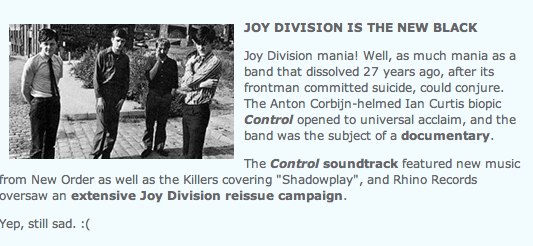In this social media excerpt against a light bluish-gray background, a black and white photograph on the left features the four young men of the band Joy Division standing on a cobblestone sidewalk with bushes behind them. They are casually dressed, with the figure on the left in a light-colored shirt and tie, the next one in a dark jacket, another in a dark shirt with his right hand raised to his face, and the last one, closer to the camera, in a light jacket with his arms crossed. To the right of the photo, bold text proclaims, "Joy Division is the new black." The article, titled "Joy Division mania," touches on the band's enduring legacy despite dissolving 27 years ago following the suicide of their frontman. It highlights the Anton Corbijn-helmed Ian Curtis biopic, "Control," which opened to universal acclaim and led to both a documentary and an extensive Joy Division reissue campaign by Rhino Records. The "Control" soundtrack included new music from New Order and a cover of "Shadowplay" by The Killers. The excerpt ends on a somber note with, "Yep, still sad," and a frowning face emoji.